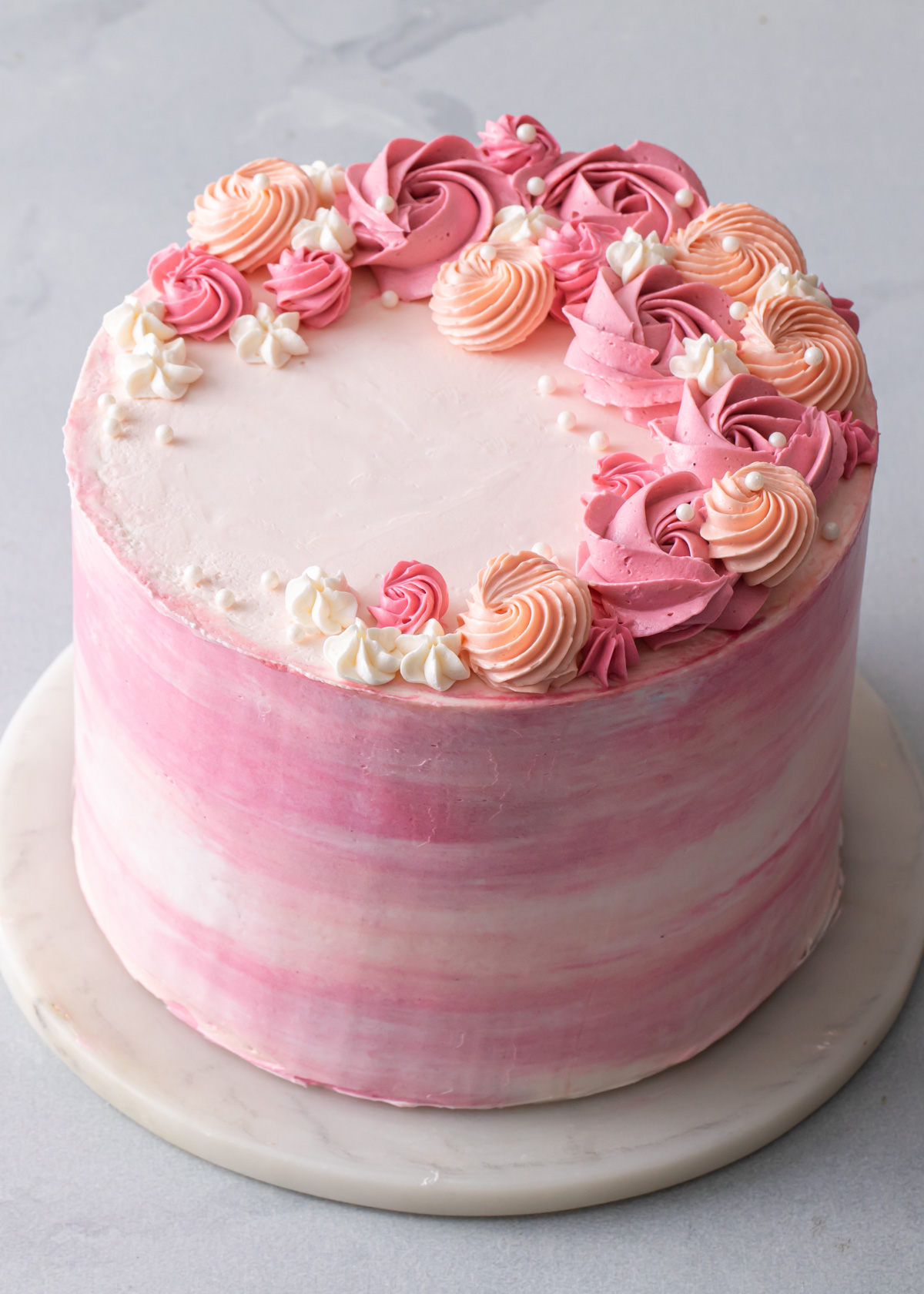This photograph showcases a beautifully decorated cylindrical cake, artistically frosted with various shades of pink and light orange, set on a round marble dish that rests on a white marble surface. The cake's sides are adorned with streaks of pinkish-white frosting, culminating in a solid, soft pink top. An elegant arrangement of pink roses, peach-colored swirls, and small white six-pointed star shapes, accented with tiny white sugar pearls, graces the upper right side of the cake, forming a crescent shape that tapers off towards the left side, leaving a portion of the white top bare. The intricate design contrasts beautifully with the simple, flat white section, highlighting the delicate craftsmanship of the sugary pearls scattered amongst the vibrant flowers.